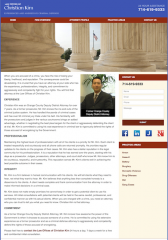**Detailed Descriptive Caption:**

The image captures a web page design with an overall vertical rectangular format. The layout is bordered on three sides—left, right, and top—with a rich royal blue hue, while the bottom edge either lacks a border or features a light gray strip. 

At the very top, a horizontal rectangular section in the same royal blue color spans across the page, featuring white text on both its left and right sides. Below this, a red horizontal band provides headings for various columns, also in white font, though the text appears very small and slightly blurry.

The main content of the web page includes an image prominently displayed horizontally. This image showcases four large, cream-colored pillars set outdoors, with the American flag visible between two of the pillars.

Beneath this imagery, text begins to populate the left side of the page. Each paragraph is followed by a new heading in black, bold font. Unfortunately, the small size renders the text unreadable.

To the right of the textual columns, there is a vertical image of a man standing with a tree in the background, accompanied by text in white at the bottom of this image. 

Further to the right, a horizontal rectangular area is presented, leading down to various white fields set against a light tan background. Towards the bottom of this column, several social media icons, including those for Facebook and LinkedIn, make an appearance. The remainder of this right-hand column continues with the light tan background, creating a cohesive visual flow.